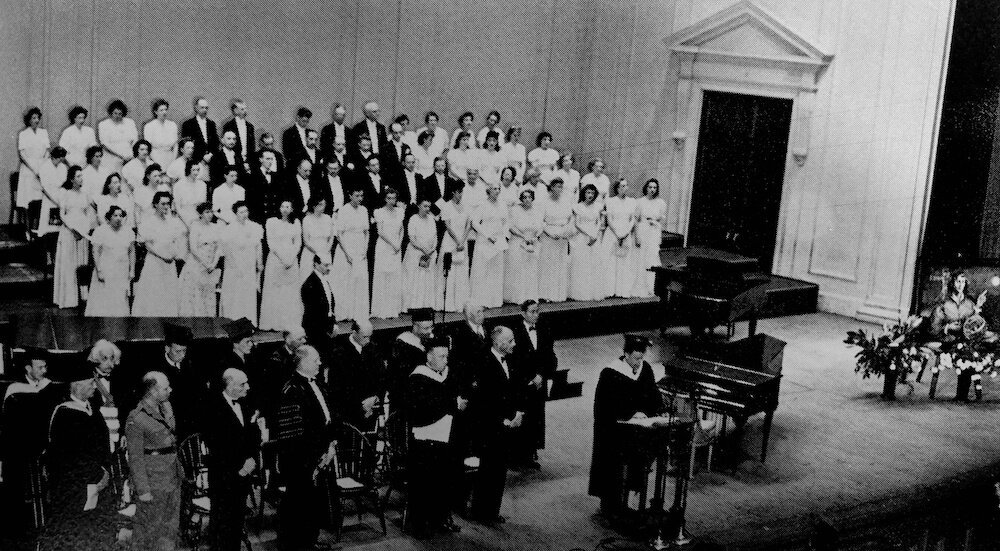This black-and-white photograph captures the interior of what might be a church or hall, set up for a formal event, possibly a graduation or commencement ceremony. Center right is a speaker in a cap and gown at a lectern, situated on a large stage. To the left of the speaker, the stage is crowded with a choir composed predominantly of 20 women in white dresses flanked by 12 men in black and white tuxedos. Below the stage, to the left side, is a group of men in formal wear, one conspicuously dressed in a soldier’s uniform, and among them, a gentleman resembling Albert Einstein, distinguished by his characteristic white hair. Also notable are two pianos positioned to the right of the lectern, one directly behind the other. Far right in the image is a painting, possibly a memorial, adorned with flowers, suggesting the event could be of a commemorative nature. The scene is meticulously captured in shades of black and white, reflecting the solemn yet celebratory atmosphere.